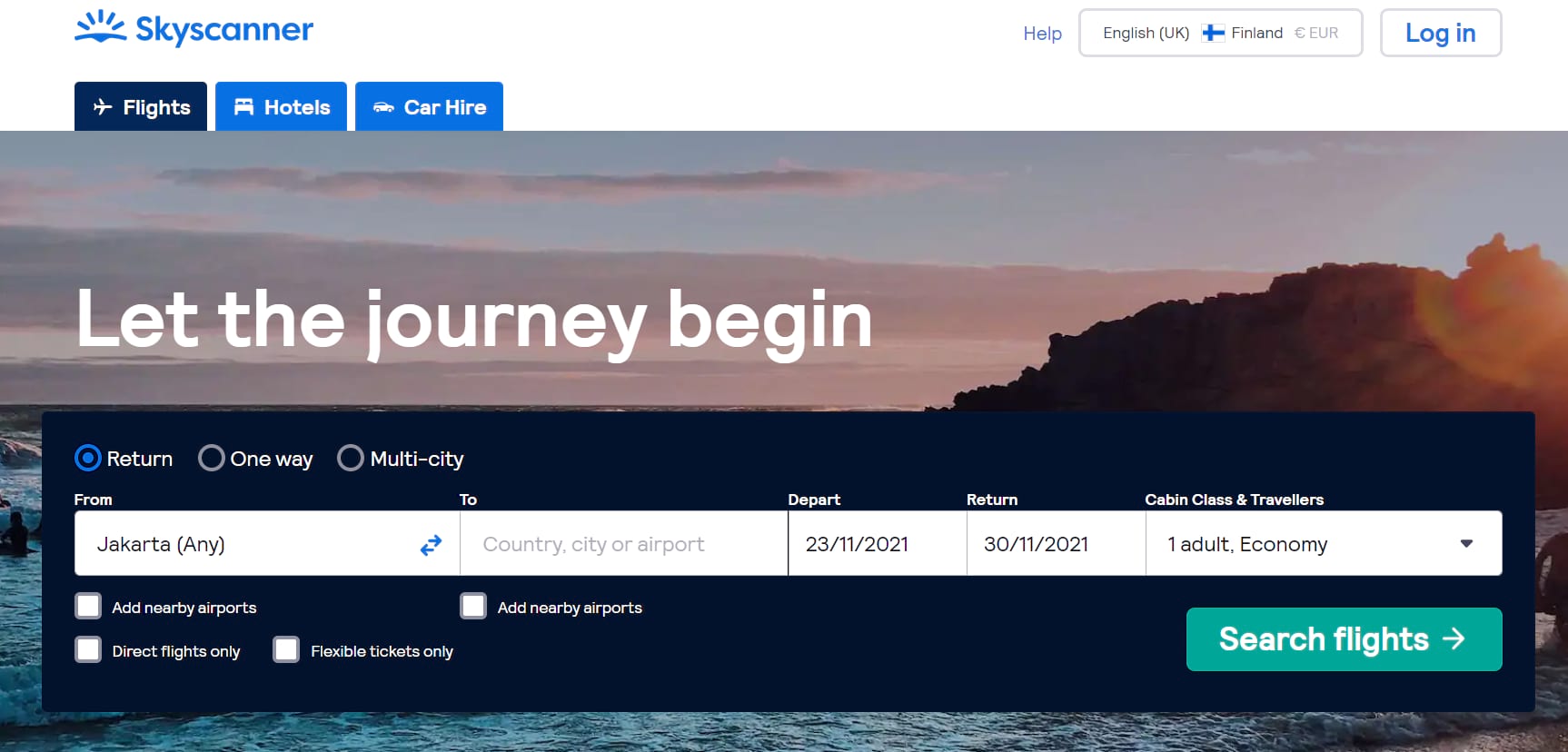Screenshot of the Business SkyScanner Web Page

In the top left corner of the screenshot, the "SkyScanner" logo is prominently displayed in a combination of dark blue and medium blue hues, positioned beside a blue sunburst horizon icon. On the far right, there's a "Help" link in blue, accompanied by a dropdown box that displays "English (UK)" and features the Finnish flag. The dropdown further includes "Finland" and the Euro symbol with "EUR" in light grey. Next to this is a "Log In" link in blue.

Directly beneath the SkyScanner logo are three tabs: "Flights," "Hotels," and "Car Hire." The "Flights" tab is highlighted with a dark blue background and features a white airplane icon, indicating it is the selected option. The "Hotels" tab has a medium blue background with a white bed icon, and the "Car Hire" tab is similarly styled with a blue background and a white car icon.

The majority of the screen showcases a large, rectangular search section. The background image is a beach scene, depicting people in and around the ocean, a nearby hill, and clouds in the sky. Superimposed on the clouds are the words "Let the journey begin" in white text. Below this text is a long search bar with three options: "Return," "One Way," and "Multi-City." The "Return" option is highlighted with a blue circle and dot.

The search bar includes several fields:
- The "From" field is filled with "Jakarta (any)" and accompanied by left and right arrows.
- The "To" field invites users to enter a country, city, or airport.
- The "Depart" field shows the date "23-11-2021."
- The "Return" field shows the date "30-11-2021."
- The "Cabin Class & Travelers" field is set to "1 adult, Economy" with a dropdown for more options.

Below these fields are four additional checkboxes for refining the search:
- "Add nearby airports" (under the "From" field)
- "Direct flights only"
- "Flexible tickets only"
- Another "Add nearby airports" checkbox (under the "To" field)

Finally, a light blue "Search Flights" button is located at the bottom right corner of the search section.